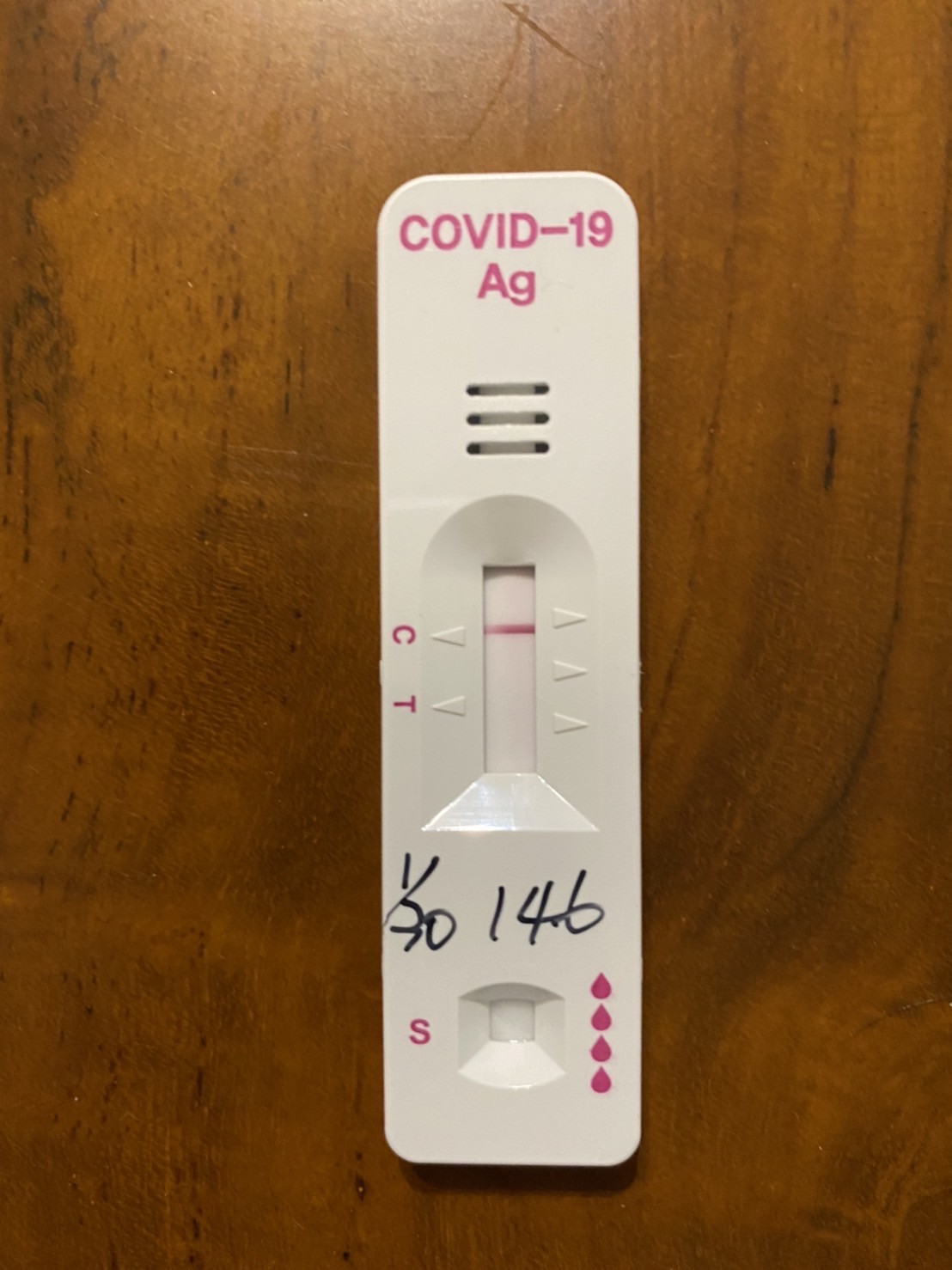This image features a COVID-19 antigen rapid test, characterized by its oblong shape and white plastic exterior. At the top of the test, the text "COVID-19" is prominently displayed in bold pink letters, with "COVID" entirely capitalized. Beneath this, a capital "A" is followed by a lowercase "g". The middle section features three horizontal slats integrated into the test.

A dome-shaped structure with a trapezoid base houses a window that displays a horizontal pink stripe. On either side of this window are two white triangles; the left triangle points to the letter "C", and the lower triangle points to a "T". Below these elements, the numbers "1-30" and "146" have been handwritten in marker.

Additionally, there is a smaller window towards the bottom left of the test, marked by a pink letter "S". To the right of this window are four droplet symbols, resembling blood droplets. The entire test rests on a brown wooden table.